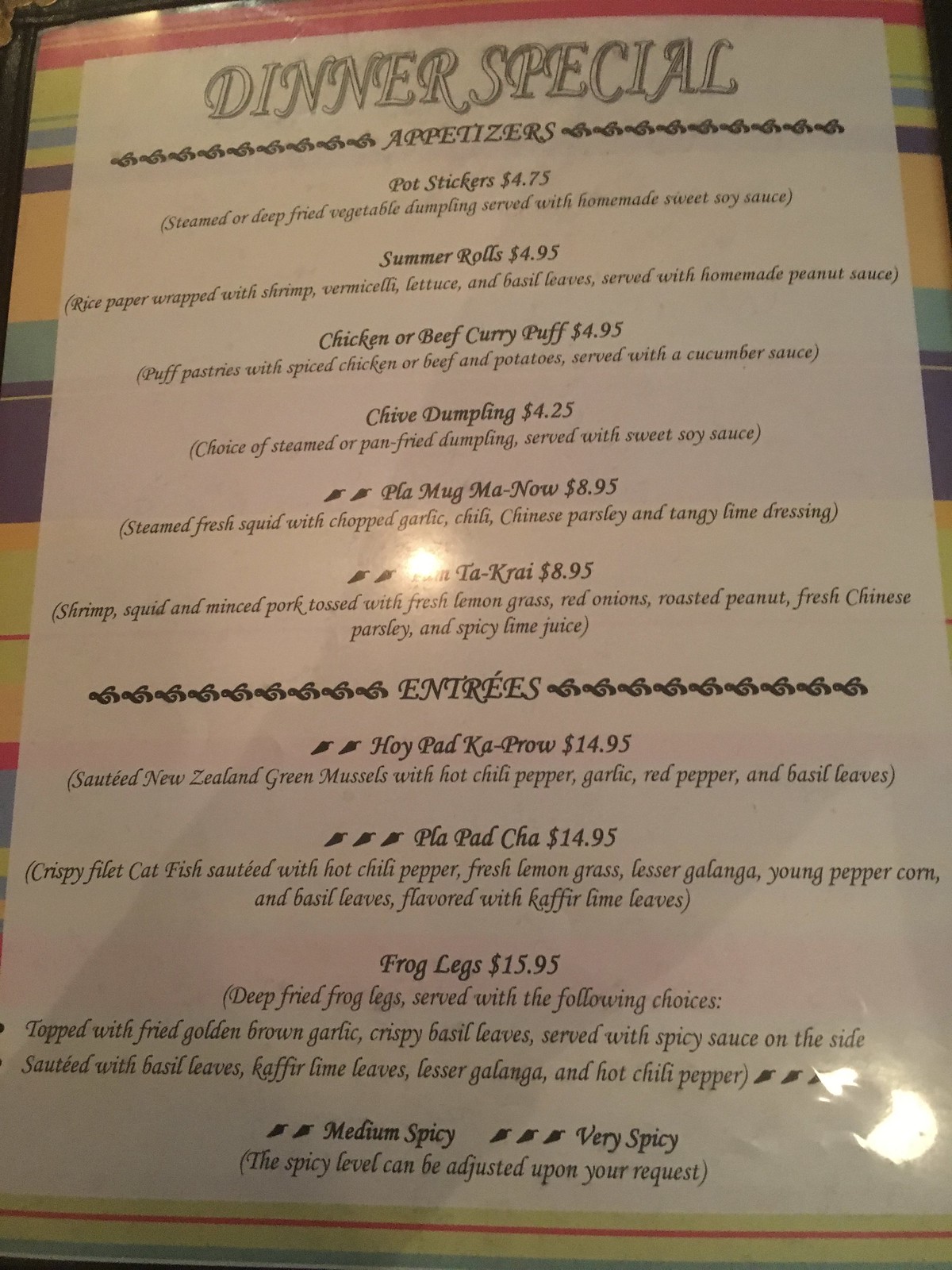Here's a detailed and cleaned-up description of the image:

The image showcases a vibrant and colorful menu with a pastel striped border in shades of pink, green, blue, orange, and purple. At the top of the menu is the heading "Dinner Specials."

### Appetizers
- **Pot Stickers - $4.75**  
  Steamed or deep-fried vegetable dumplings served with homemade sweet soy sauce.
- **Summer Rolls - $4.95**  
  Rice paper wrapped with shrimp, vermicelli, lettuce, and basil leaves, served with homemade peanut sauce.
- **Chicken or Beef Curry Puff - $4.95**  
  Puff pastries filled with spiced chicken or beef and potatoes, served with cucumber.
- **Chive Dumpling - $4.25**  
  Choice of steamed or pan-fried dumpling served with sweet soy sauce.
- **Pla Mug Manao - $8.95**  
  Steamed fresh squid with chopped garlic, chili, Chinese parsley, and tangy lime dressing.

### Entrees
- **Hoi Pod Kai Prow - $14.95**  
  Medium spicy (indicated by two peppers) dish.
- **Pla Pad Sam - $14.95**  
- **Frog Legs - $15.95**  
  Very spicy (indicated by three peppers) dish.

This menu captures the essence of a diverse and flavorful dining experience with a range of appetizers and entrees.